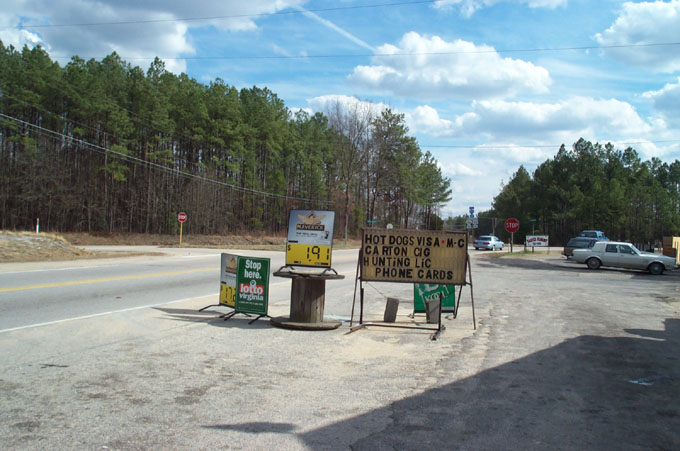This vibrant photograph depicts an exterior scene of a rural convenience store, likely positioned along a lesser-traveled national road, perhaps near a national park or holiday destination in the state of Virginia. The day is bright and sunny, with a baby blue sky populated by an abundance of fluffy white clouds. The setting is surrounded by clusters of pine trees lining both sides of the road, enhancing the countryside atmosphere.

Prominently in the middle of the image are a few signs, one of which is green and reads "Stop Here Lotto Virginia." Beside it, another sign on a stool reads “$1.91,” though additional details are unclear. A larger, weathered yellow sign changes its message using black letters, advertising "Hot Dogs, Visa, MC, Cotton, Cigarettes, Hunting Lic, and Phone Cards."

The store appears to have a concrete forecourt extending to the road, marked by a yellow double center line. A stop sign and several vehicles—an older car close by and another driving away in the distance—are visible. A shadow cast on the right bottom edge of the photo indicates the presence of a nearby building, though the building itself is out of the frame. The scene evokes a quaint and serene atmosphere, characteristic of rural Virginia.